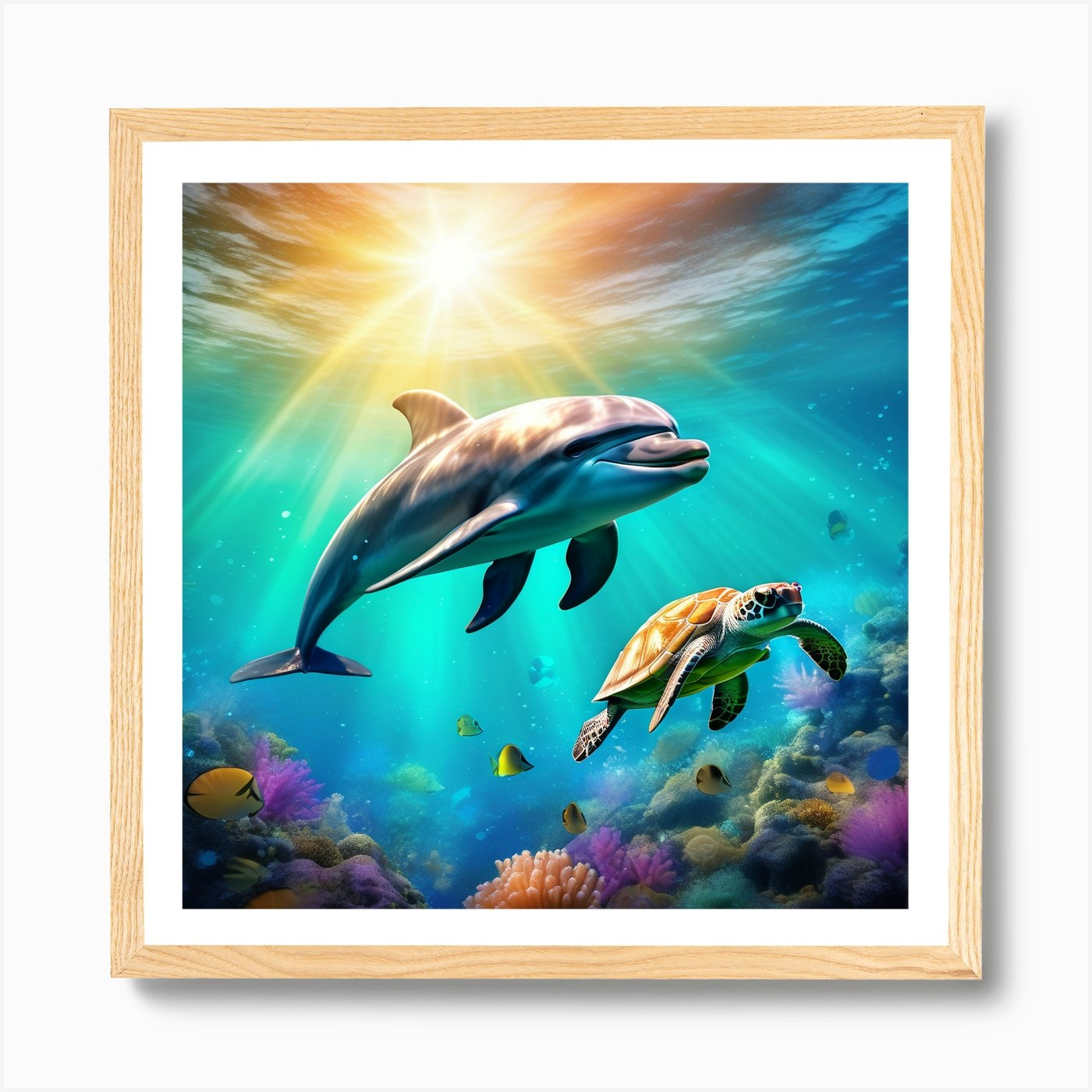This detailed image portrays a vivid underwater scene featuring a dolphin and a sea turtle swimming harmoniously side by side, their bodies angled from the lower left to the top right corner. Captured either as a highly realistic painting or an impeccably clear photograph, the setting emanates an ethereal beauty under the turquoise water. Sunlight penetrates the surface, casting warm orange and yellow beams that illuminate the dolphin, which has a gray body with a top fin, tail, and side fins. The sea turtle, boasting gray legs and head with a brown shell, glides gracefully alongside.

The bottom of this enchanting aquatic tableau is adorned with diverse coral formations in vibrant shades of purple, pink, green, yellow, and orange. Some of the corals are peachy and magenta purple, interspersed with various sea plants and small yellow fish, adding more life and color to the scene. Bubbles float towards the top right corner, merging into the blue sky visible at the water's surface where the sun's rays originate. Framed in a light beige wooden frame, the image's indoor setting contrasts with the depicted outdoor underwater world, bringing a touch of marine tranquility into the living space.